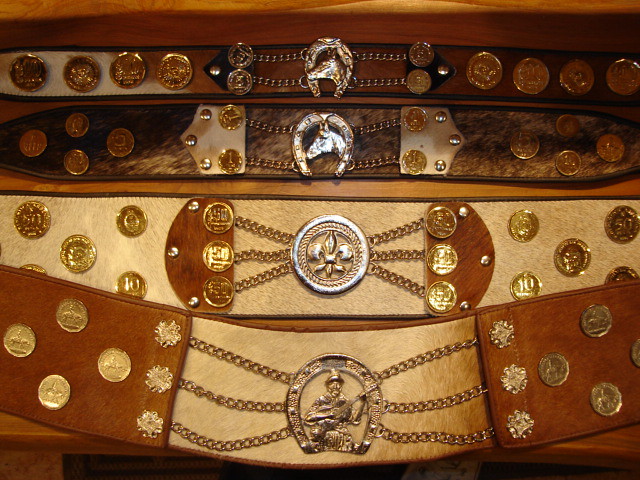This image showcases four ornate, decorative belts arranged horizontally across a brown wooden table. The belts are positioned with the narrowest at the top and the widest at the bottom, nearly touching one another, with the bottom belt slightly overlapping the one above. Each belt features a central medallion from which chains extend to circular coin-like decorations on either side. The design of the medallions varies: the top two belts have an upside-down horseshoe with a horse's head, the third belt displays a roped-edge circle with a fleur-de-lis, and the bottom belt features an upside-down horseshoe with a man holding a rifle. The belts, crafted from varying leathers, range in color from dark brown to tan and are studded with intricate, metallic details. A leg of the brown wooden table is partially visible in the bottom left of the image, adding context to the setting of these elaborately designed belts.